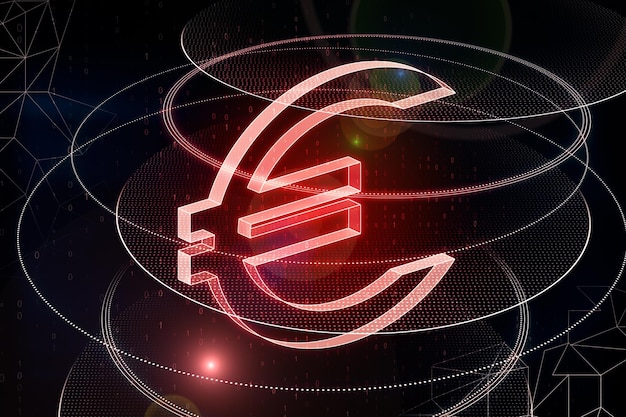The image showcases a striking, luminescent Euro (€) symbol at its center, glowing in vibrant red. The symbol itself appears to be transparent in parts, blending seamlessly with the black background. Surrounding the Euro symbol are multiple layers of white circles, creating a visually dynamic, almost 3D appearance. Flanking the central icon, at the bottom right and top left corners, are clusters of various polygonal shapes, adding to the graphic complexity. Additionally, the left side below the Euro symbol features more red lighting effects, contributing to the overall glow. Subtle, almost hidden within the background, are sequences of numbers that suggest a coded or digital element, enhancing the modern, tech-inspired aesthetic of the piece.